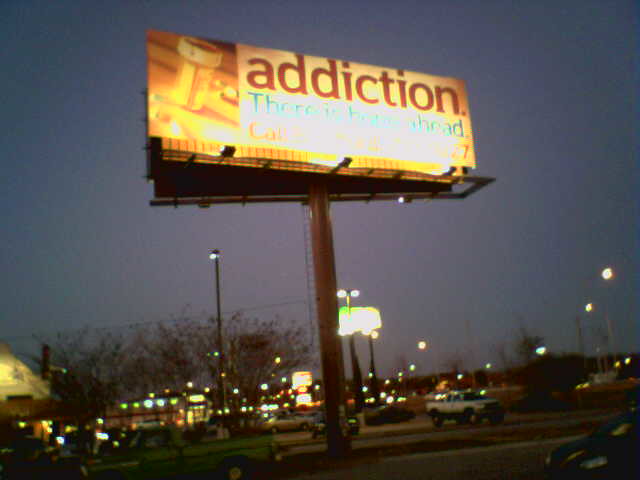In this urban twilight scene, a prominent billboard stands against a dusky blue sky on the cusp of sunset. The billboard reads "Addiction" in a brownish font, with a backlight that makes it challenging to discern the exact color. Adjacent to the word "Addiction," an image of a pill bottle with pills spilling out adds to the impactful message. Below the word "Addiction," partially obscured by a bright highlight, the phrase "ahead" can be faintly read, implying a cautionary message. The city's ambient lights have started to flicker on, illuminating buildings in the background. Streetlights cast a warm glow over the the bustling street below, where a white pickup truck and a gray car are among the vehicles navigating the evening traffic.